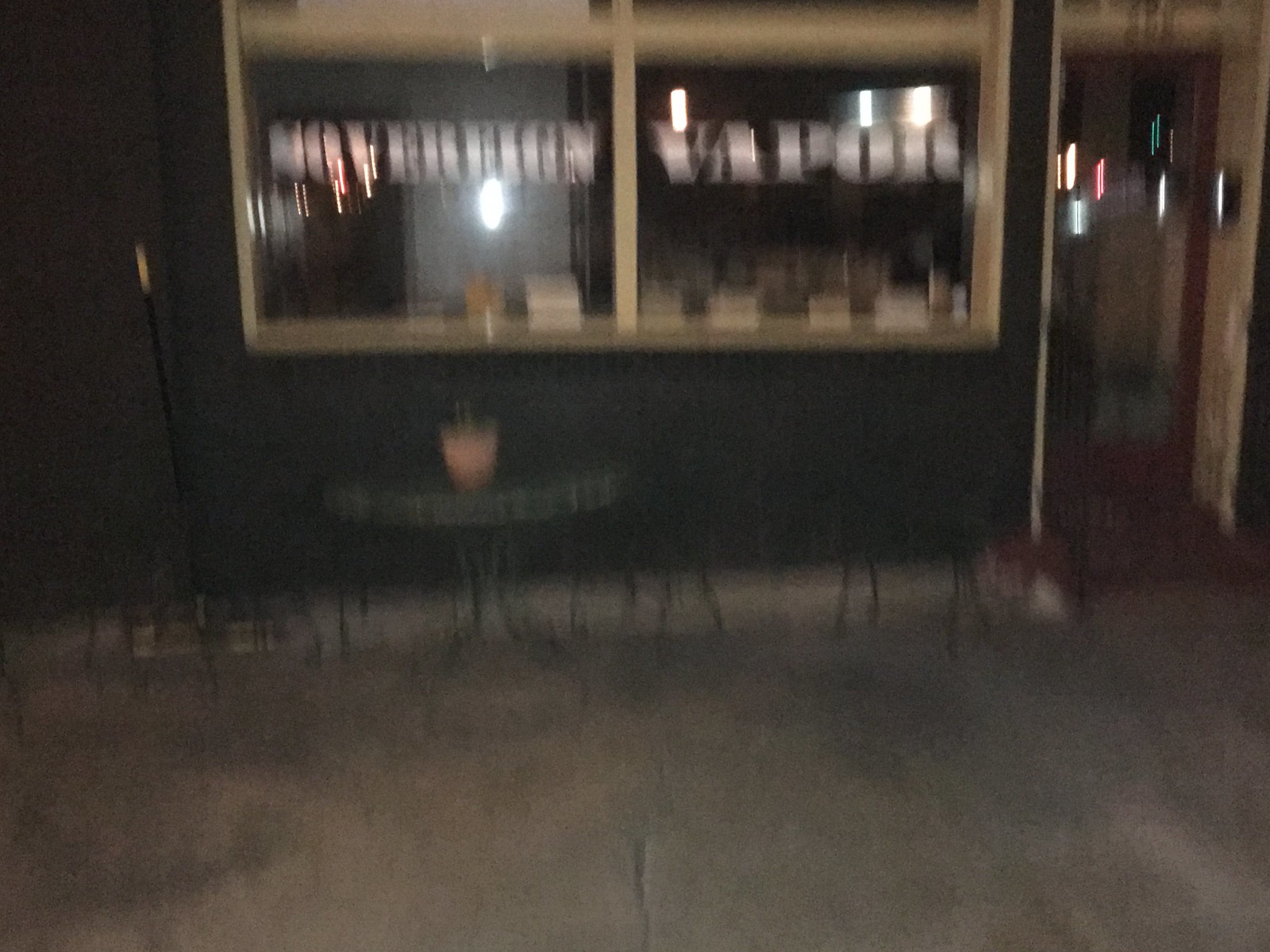A blurry nighttime image depicts the front facade of a business with two large windows. Despite the lack of clarity, the storefront is identifiable as "Sovereign Vapor," with "Sovereign" displayed in white font on the left window and "Vapor" on the right window. The business features a whitish-tannish window frame. In front of the window with the "Sovereign" sign, there is a round metal table. The building facade appears to be green, and the entrance door is situated on the right side of the image.